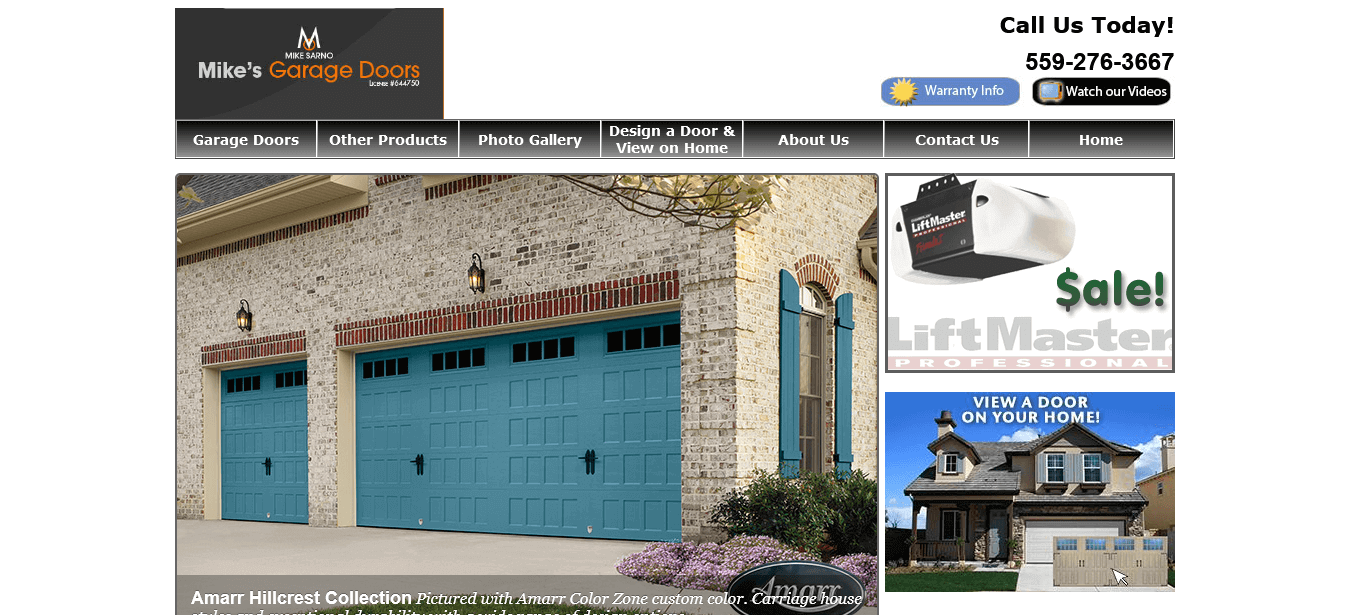This advertisement from Mike's Garage Doors features a sleek, professional layout on a black background with a large, prominent "M" above an inviting garage entrance. The company name is presented in white text, while "Garage Doors" is accentuated in orange for a visually striking contrast. The call-to-action "Call us today" directs viewers to a specified phone number, under which "warranty info" is noted for customer assurance. 

A large sun graphic adds a cheerful touch, guiding viewers to watch various videos available through a clickable link. Navigation headers are displayed in dark gray boxes, offering quick access to "Garage Doors," "Other Products," "Photo Gallery," "Design a Door," "About Us," "Contact Us," and "Home."

Beneath these options lies an expansive image of an elegant, tan brick house featuring vibrant turquoise garage doors from the Amar Hillcrest Collection. The property boasts one single garage door and two double doors side-by-side.

Adjacent to this main image are two smaller boxes. One highlights a LiftMaster garage door opener, clearly marked with a green "Sale" label. The other invites users to "view a door on your home," showcasing a brown-toned house with a driveway and a superimposed image of tan garage doors, demonstrating the aesthetic appeal and customization options available.

Overall, this detailed advertisement effectively combines essential product information, customer engagement elements, and intuitive navigation to offer a comprehensive overview of Mike's Garage Doors' offerings.